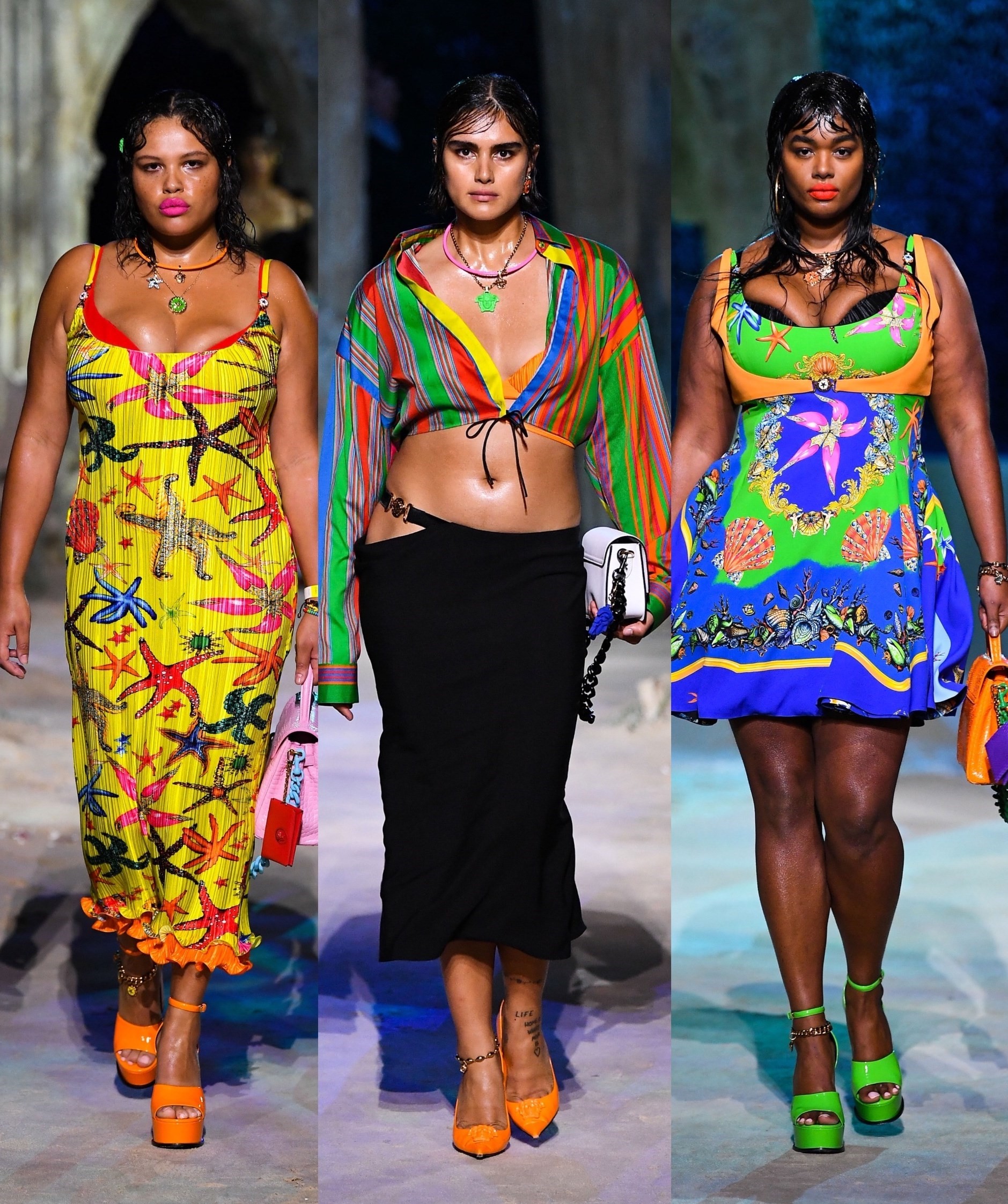This image features a split-screen composition showcasing three models, each wearing vibrant and colorful outfits, walking down a fashion runway. On the far right, a black woman is elegantly clad in a bright, summery dress with a blue and green skirt and a top infused with orange and green hues. Completing her look are eye-catching green platform shoes. In the center, a Hispanic woman dons a striking ensemble with a black calf-length skirt that hangs gracefully to the side, paired with a striped, multi-colored crop top tied at the breasts, revealing an orange bra underneath. She accessorizes with pointed orange heels. On the left, another black woman walks confidently in a bright yellow dress adorned with starfish patterns that nearly reaches her ankles, accompanied by bold orange platform shoes. Her look is accentuated by her bright pink lipstick, bringing a vivid pop of color to her overall appearance.